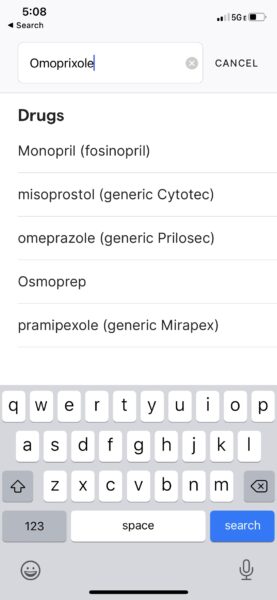This detailed caption describes a screenshot of an Android phone interface and its contents with precise clarity:

---

A screenshot of an Android phone interface. The dimensions suggest a typical phone screen, being both long and wide. In the top left corner, the time is displayed as "5:08." On the top right, there are indicators for the phone's status, including two signal bars, a "5G" network symbol, and a battery icon showing slightly less than halfway charged. Directly below this row of indicators, from left to right, is a back arrow icon labeled "Search." 

In the search bar below, text reads "OmoPrixole," followed by a small "X" inside a box, with the label "Cancel" situated outside the search box. A thin line demarcates this search section from the content below. 

The next section displays a header with the word "Drugs" in bold on the left-hand side. Below this header, "Monopril (Fosinopril)" is listed, with "Fosinopril" indicated in parentheses as an alternative name. There are additional entries under this category, amounting to a total of five selections. 

Finally, at the very bottom of the screen, a keyboard interface is visible, indicating that the user can enter text.

---

This caption provides a thoroughly detailed description of the screenshot, encapsulating all visible elements and their arrangement on the screen.